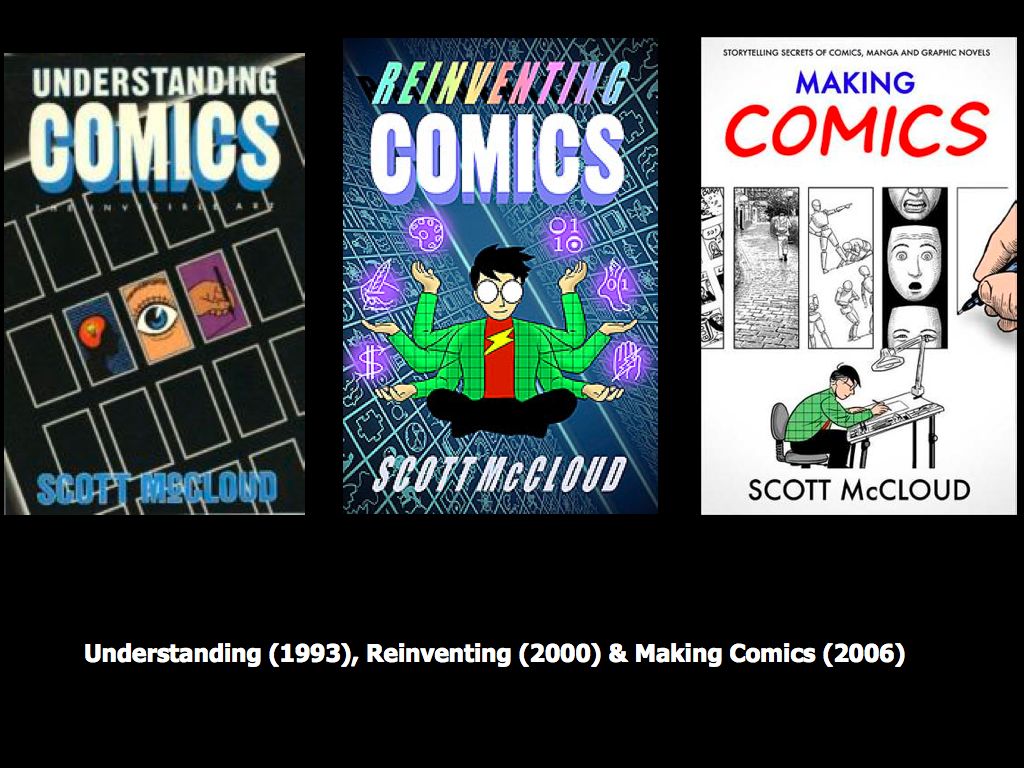The image features the covers of three books by Scott McCloud, set against a black background. The leftmost cover is titled "Understanding Comics" and depicts a series of rectangles with various illustrations: an eye, a hand holding a pencil, and a thought bubble with a lit light bulb. The author's name, Scott McCloud, is at the bottom. The center cover, "Reinventing Comics," displays an animated image of a man seated in a meditative yoga pose with six arms, each arm holding different symbols. The man wears a green jacket over a red t-shirt with a yellow lightning bolt, has black hair, and large glasses. Scott McCloud's name appears again at the bottom. The rightmost cover, titled "Storytelling Secrets of Comics, Manga, and Graphic Novels," with a subtitle of "Making Comics," features a white background with several black-and-white comic panels showing diverse faces and a man in a green shirt at a drawing desk. The name Scott McCloud is also at the bottom. Below these three covers, text contextualizes their publication years: "Understanding 1993, Reinventing 2000, and Making Comics 2006."